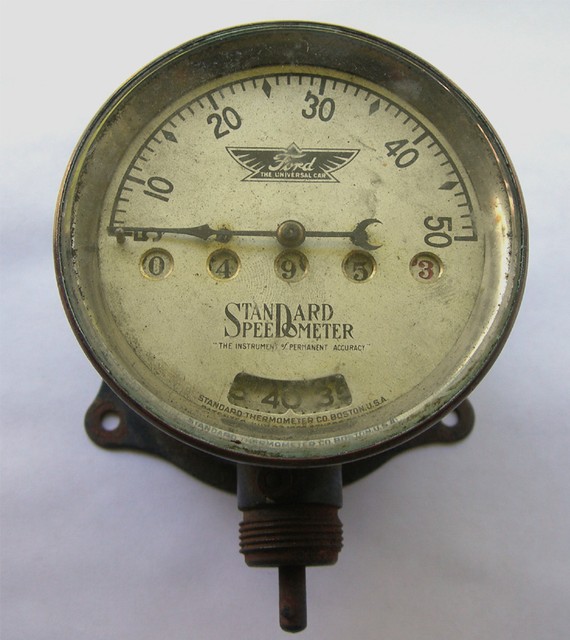This photograph showcases a beautifully preserved antique speedometer, originating from a very old vehicle. The speedometer, crafted by the Standard Thermometer Company in Boston, USA, features an analog dial where the top speed indication is 50 mph—a speed that this early automobile likely never achieved. The odometer reads 49.53 miles, without tenths of a mile indicated, emphasizing its age and the period's technological limitations.

The dial prominently displays the "Ford, the Universal Car" logo above its analog pointer, marking it as an authentic piece from the legendary auto manufacturer’s early days. The speedometer is encased in a chrome or metal bezel, complete with a threaded attachment point, screw holes, and a mounting flange on the back. This threaded area would connect to a rotating cable sheathed and routed to the vehicle's wheel or another below-engine connection point.

This meticulously detailed and historically significant speedometer, hailing from the early 20th century, is not just an instrument of permanent accuracy but also a testament to the humble beginnings of automotive engineering.